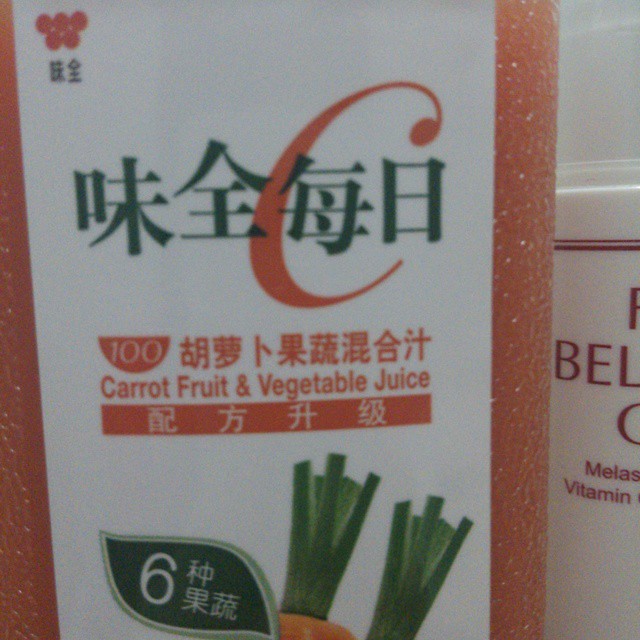This is a close-up photograph of a vibrant orange bottle of carrot fruit and vegetable juice featuring a bilingual label in both English and an Asian script, possibly Japanese or Chinese. Dominating the image is the brand name in large characters with a prominent "C" and a graphic of an orange cutting across the lettering. Below that, the words "carrot fruit and vegetable juice" are clearly printed. There is an orange strip with white writing in the Asian script beneath this. At the bottom of the label, a small tag featuring the number six is visible alongside additional Asian characters, likely detailing nutritional information. You can see the tops and partial bodies of carrots, reinforcing the juice's primary ingredient. The bottle is frozen on one side, suggesting it is stored in a refrigerator, and next to it is another container, white in color, with partially visible red lettering that includes the letters "B-E-L" and the word "vitamin." The overall setting appears to be a refrigerated display, emphasizing the freshness of the juice.